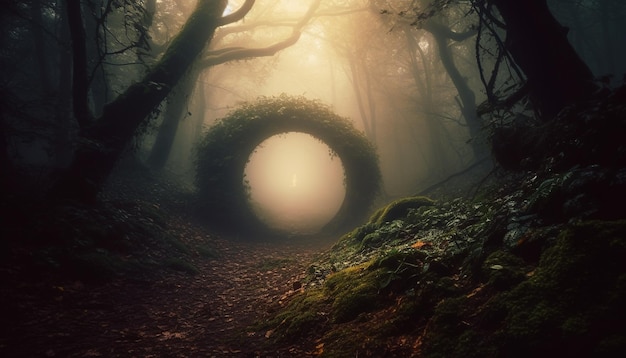The image is a photorealistic, digitally created scene set in a dark, dense forest. It features tall, silhouetted trees flanking both sides of the composition, which fade into a foggy, white background illuminated by diffused sunlight. The forest floor is scattered with dead leaves, moss-covered boulders, and tree roots, creating a somewhat eerie ambiance. The focal point of the image is a nearly perfect circular structure in the middle, possibly a moss-covered log or a gateway made of leaves. This circular ring stands at the center of an elevated path, inviting the viewer into the fog-enshrouded distance. The overall tone of the scene is soft and somewhat blurry, contributing to the mysterious and surreal atmosphere.